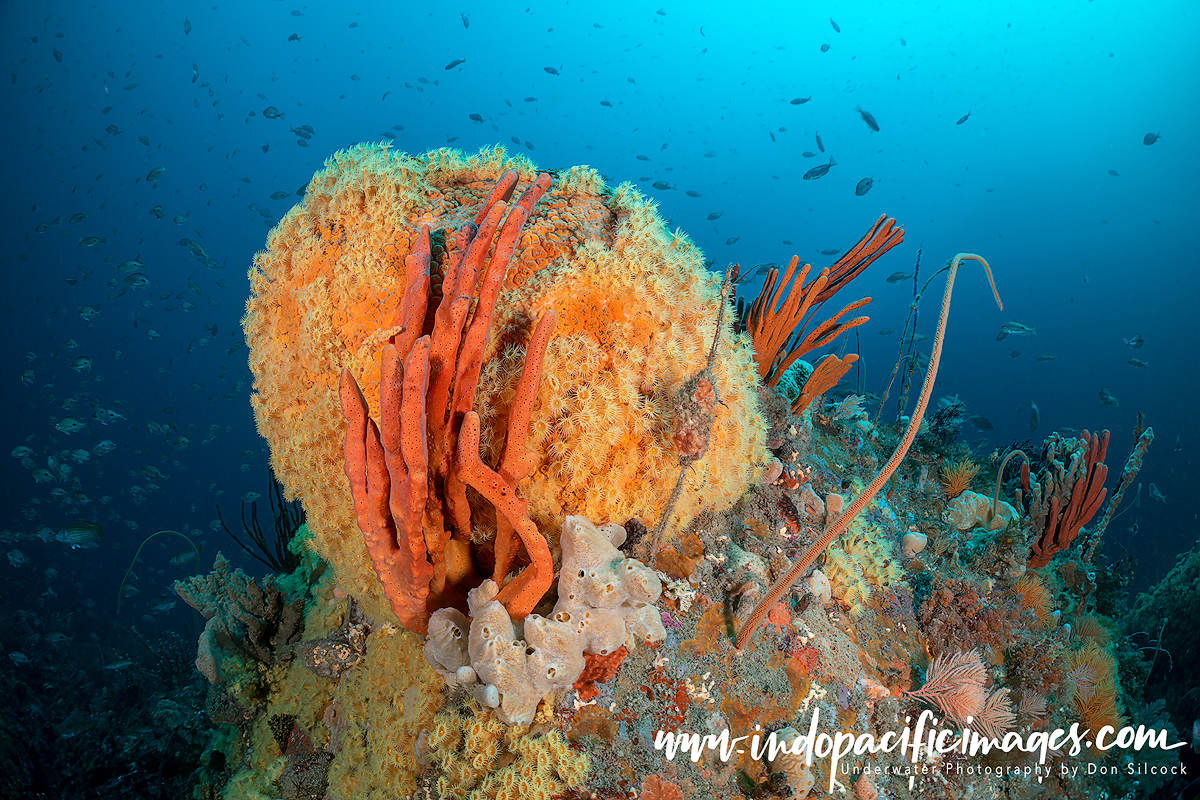This highly detailed underwater photograph captures a vibrant coral reef immersed in an oceanic backdrop. The background showcases a gradient of blues, fading from a bright, almost turquoise hue in the top left to a deep navy blue at the bottom left, representing varying depths and light penetration. Surrounding the coral reef, numerous small fish, likely hundreds, create a dynamic flurry of activity, their silver bodies glinting as they swim in schools throughout the image.

The reef itself is anchored in the foreground by a boulder teeming with an array of colorful corals. The corals exhibit a stunning palette ranging from burnt orange and yellow to green and pink, each variety with unique shapes and textures. Some corals extend like delicate, wispy fronds, others resemble fingers or floral pockets, while some are distinctly spongy with overlapping patterns. Dominant in this vibrant reef composition is a large light orange coral adorned with white circular formations that exhibit tiny leg-like structures, juxtaposed with dark orange fronds.

In the bottom right corner, the image bears a professional touch with a watermark that reads "www.indopacificimages.com" in an elegant cursive script, followed by "Underwater Photography by Dawn Silcock" in a more formal font, affirming the artistry and expertise behind this captivating scene.